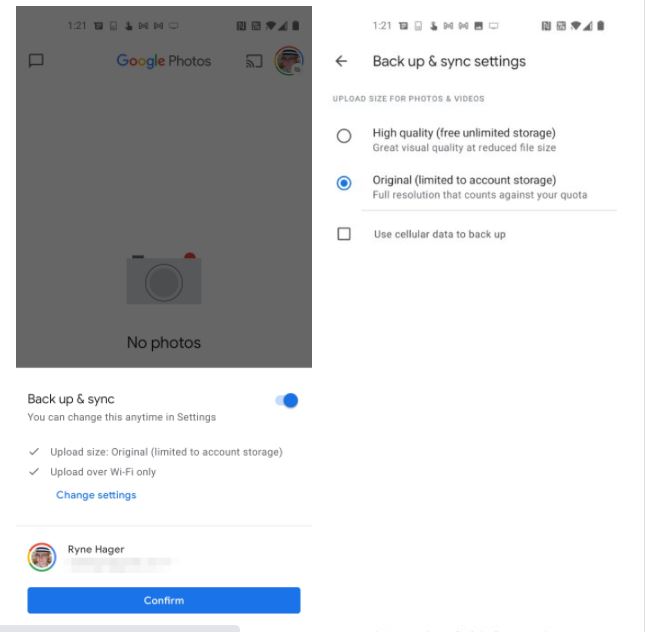A Google Photos screen is displayed, predominantly grayed out, with various settings and options visible. At the top, the number "121" is indicated. There are messaging options and the recognizable Google Photos logo, featuring the colorful Google lettering in red, green, blue, and yellow. The interface includes icons for messaging, a camera, and a profile image.

Beneath the main header, the screen shows "Backup and Sync Settings" on the right, accompanied by a back arrow for navigation. Under this section, users can select the upload size for photos and videos. The options include "High quality" with free unlimited storage and reduced file size, and "Original," which is highlighted in blue. The "Original" setting offers full-resolution uploads but is limited to account storage and counts against the quota.

Further down, there's an unchecked option labeled “Use cellular data to backup.” Below this, the text explains that "Backup and sync" can be altered in settings. Current settings indicate that "Backup and Sync" is enabled, the upload size is set to "Original,” and uploads are allowed over Wi-Fi only, which is also checked. 

At the bottom of the screen, there is an area displaying the user's profile information - "Ryan Hagarin" with a profile picture beside a blue "Confirm" button.